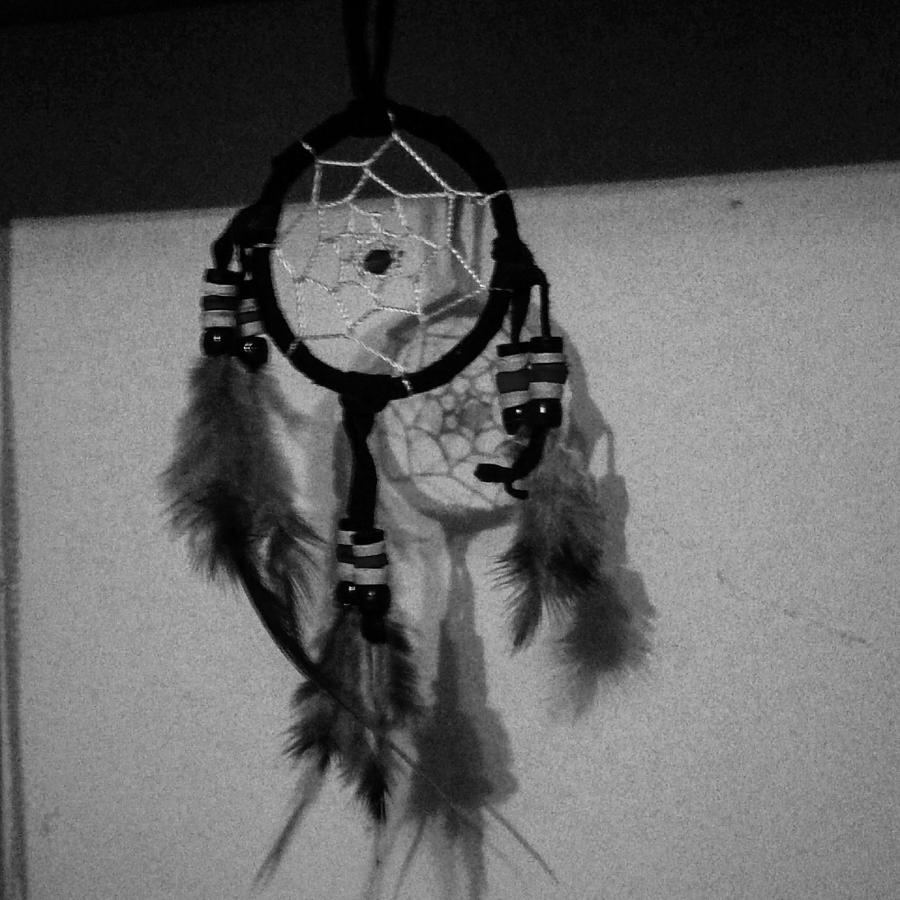This black-and-white photograph captures a dreamcatcher hanging against a wall, with its shadow cast a few inches behind it. The dreamcatcher, predominantly black in this monochromatic image, features a central circle adorned with a spiderweb-like weaving, possibly made of rope. Around this central web, white and gray beads add texture and contrast. Hanging from the bottom and sides of the dreamcatcher are three sets of leather straps, each embellished with beads and culminating in long, gray feathers. The image suggests the dreamcatcher is more of a decorative item than an authentic artifact, yet its intricate details and shadow create a compelling visual.